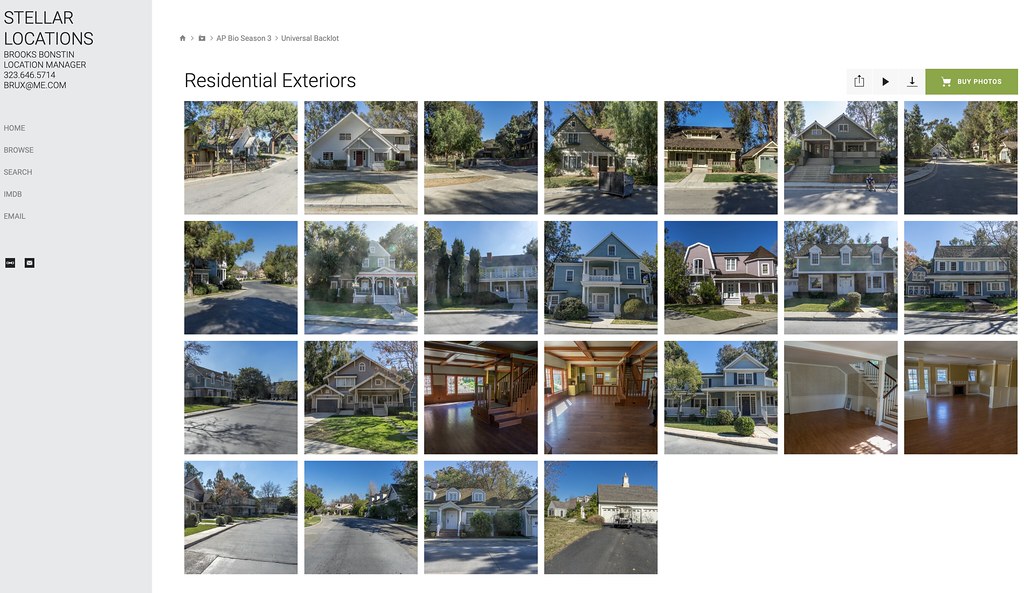The image is a horizontally rectangular screen grab from a website. On the left side, there is a narrow, vertically rectangular gray column. At the top of this column, "Stellar Locations" is written in black, followed by "Brooks Bonston, Location Manager" and a contact number, "323-646-5714." Below that, an email address, "BRUX@me.com," is listed. Beneath the contact information, there is a vertical menu with tabs labeled "Home," "Browse," "Search," "IMDB," and "Email."

The remaining portion of the frame features a collage of images showcasing residential exteriors, indicated by the title "Residential Exteriors" at the top. On the right side of the frame, next to the collage, there are several icons including an upload icon, a forward icon, a download icon, and a "Buy Photos" option.